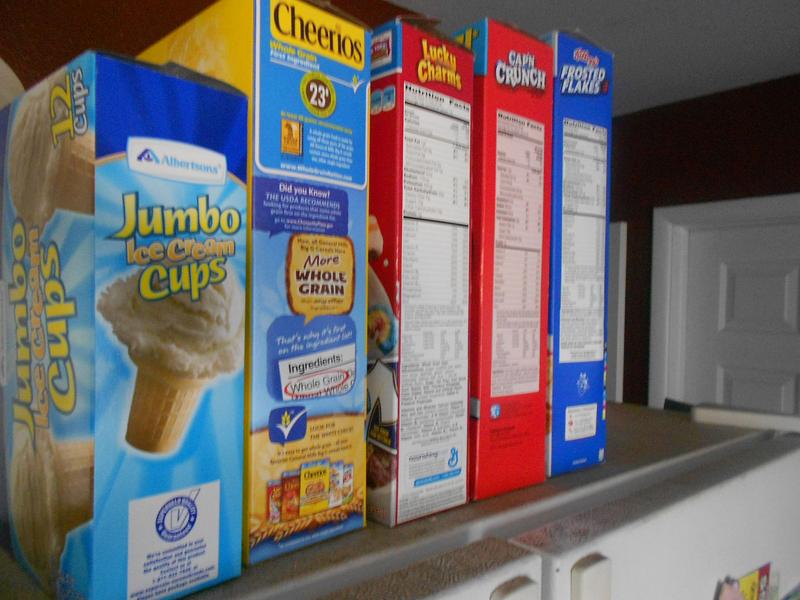In the image, on the left-hand side, there is a box labeled "Jumbo Ice Creams" featuring an illustration of an ice cream cone with vanilla ice cream in a brown waffle cone. At the bottom of the box, there is a white square containing text, and a small blue circle with the letter "V" inside it. Adjacent to this, in yellow text, the box reads "Jumbo Cups." At the top right corner, it states "12 Cups" and "Albertsons."

Next to the ice cream box, there is a box of Cheerios cereal. The side of the Cheerios box contains various information squares with text, including the number 23 at the top. In the center of the box, it highlights "More Whole Grain." Another section labeled "Ingredients" and featuring a yellow square is also visible.

Adjacent to the Cheerios box, there is a box of Lucky Charms cereal, which is red and displays "Nutrition Facts." Following this, there is a red box of Cap'n Crunch cereal, also featuring "Nutrition Facts." Finally, a blue box labeled "Frosted Flakes" (or "Killer Frosted Flakes") is visible, with its "Nutrition Facts" section contained in a white square. 

All of these boxes are placed on top of what appears to be a refrigerator. In the background, a white door and a white ceiling are visible.